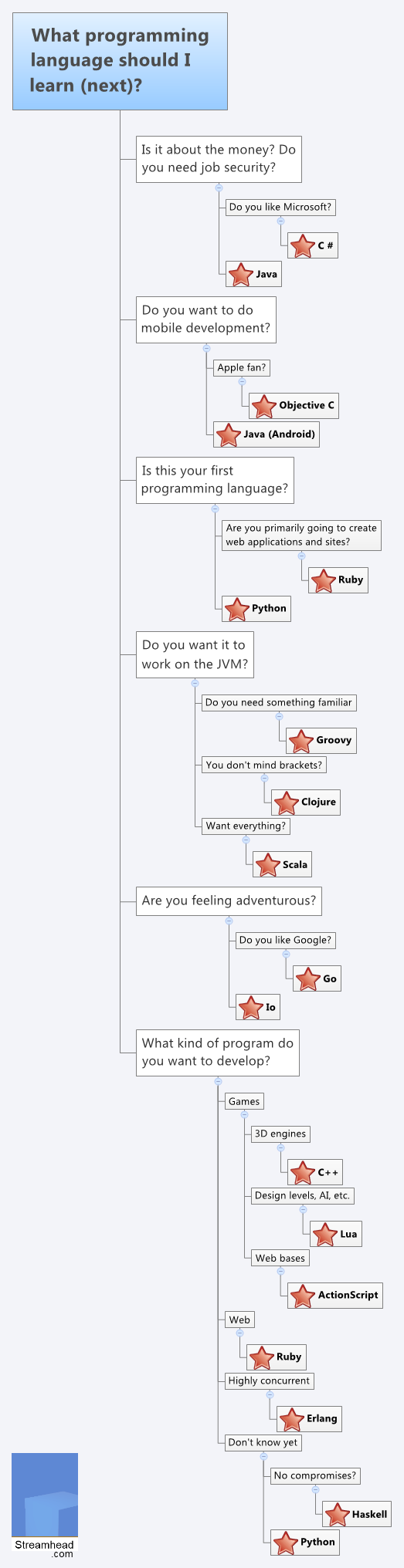This image is a screenshot of a decision-making flowchart designed to help individuals choose the next programming language to learn. The flowchart is titled, "What programming language should I learn next?" displayed in black text within a blue rectangle located in the upper left corner. The flow proceeds through a series of gray boxes with black text on a white background, each asking various questions to guide the user.

1. The first question asks, "Is it about the money?"
2. Followed by, "Do you need job security?"
3. Then, "Do you like Microsoft, Java, and C?"
4. Next, "Do you want to do mobile development?" leading to options such as "Apple Fan," "Objective C," "Java," and "Android."

The flowchart then moves on to:
5. "Is this your first programming language?"
6. "Are you primarily going to create web applications and sites?" leading to options like "Ruby" and "Python."

Further down:
7. "Do you want to work on the JVM?" with subsequent choices:
   - "Do you need something familiar?" leading to "Groovy,"
   - "You don't mind brackets?" leading to "Clojure,"
   - "Want everything?" leading to "Scala,"
   - "Are you feeling adventurous?"

Lastly, there are questions on preferences:
8. "Do you like Google?"
9. "What kind of program do you want to develop?"

In the lower left corner of the flowchart, the website StreamHedge.com is displayed in black text within a blue rectangle, identifying the source of the flowchart.